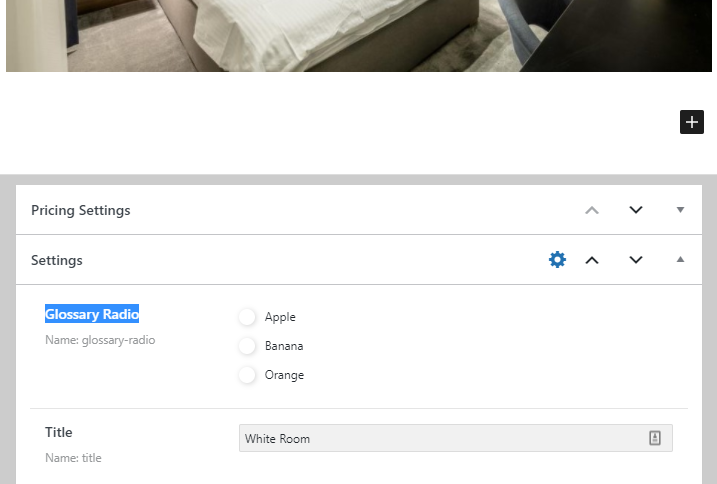In the top section of the web page snapshot, a partial, narrow rectangular image suggests the corner of a bed, possibly hinting at a hotel or shopping website. Below this image, a light gray-outlined dialog box appears, designated as the "Pricing Settings" menu. Further down, the "Settings" option is visible, followed by a highlighted blue tab labeled "Glossary Radio." This tab offers three selectable options: apple, banana, or orange. Beneath this tab, there is another submenu titled "Title," which includes a dropdown box currently set to "White Room." Overall, the page lacks sufficient context to provide a clear understanding of its purpose.